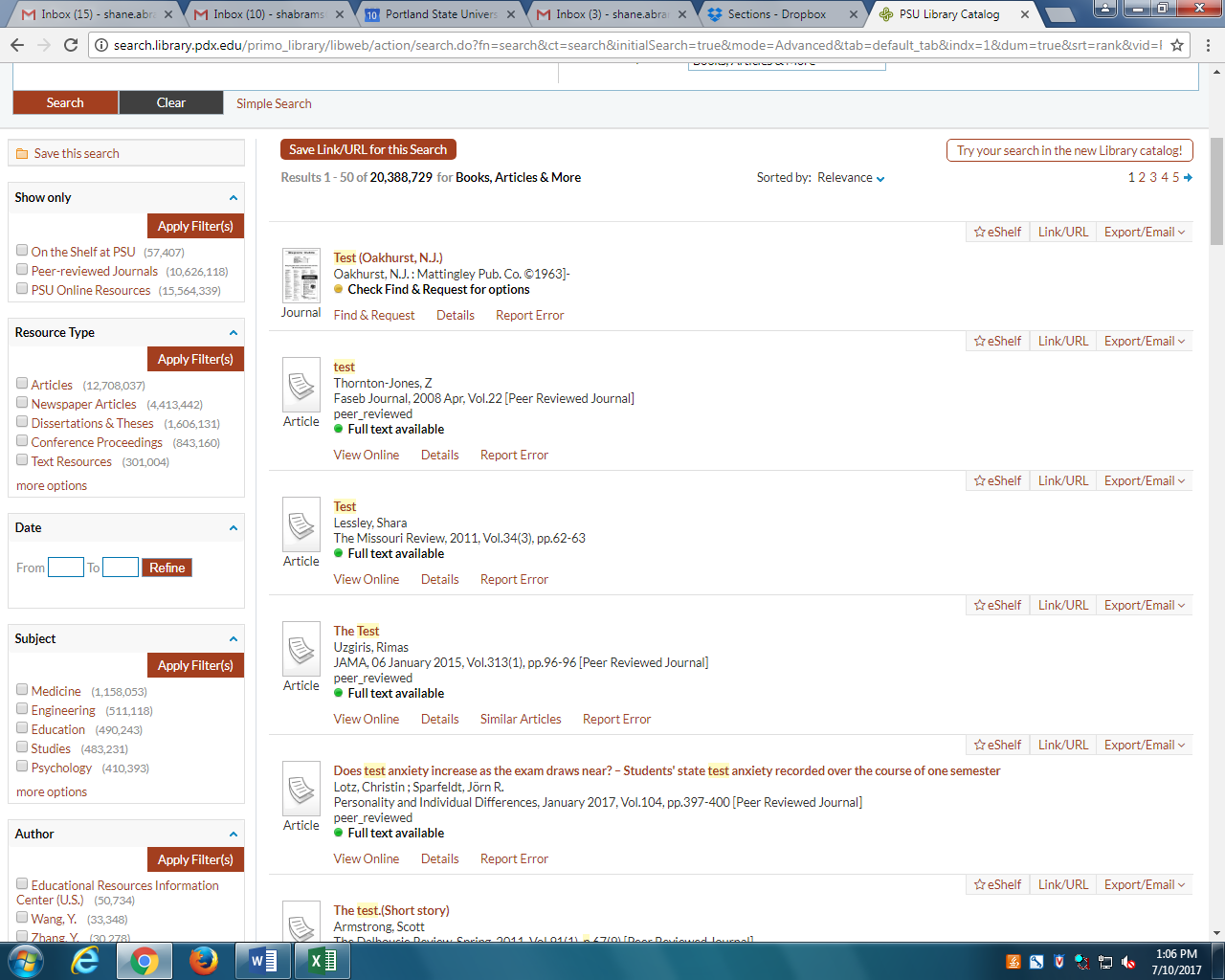This image depicts a webpage of a digital library catalog, possibly from Penn State University (PSU). The platform offers downloadable versions of various documents, including tests, articles, and books, aimed at assisting students and researchers. The interface includes a search bar which facilitates easy navigation through the extensive collection of free resources. This online library serves as a convenient tool for accessing study materials and scholarly articles remotely, enabling users to obtain PDFs of essential academic documents without having to visit the physical library.